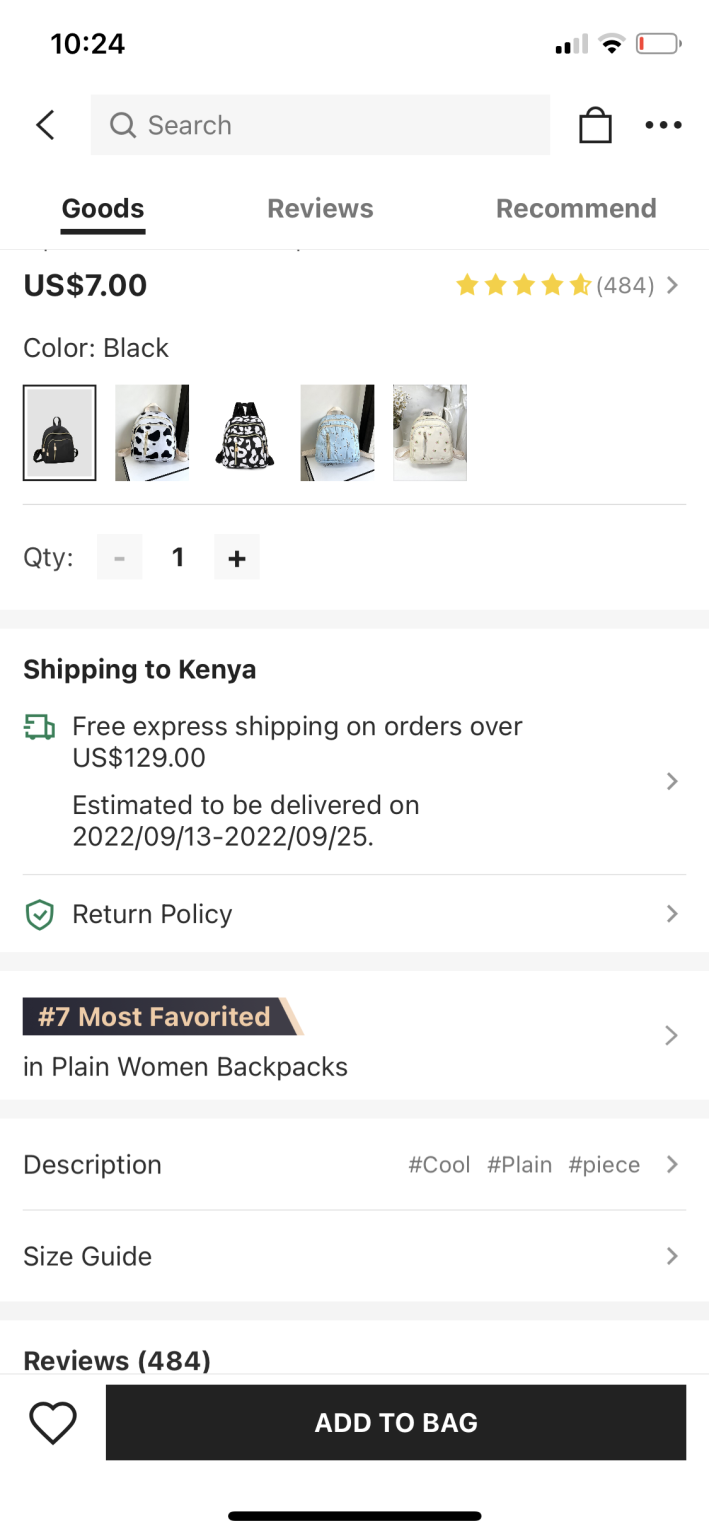Screenshot from a mobile device showing the timestamp at 10:24 AM with two bars of cellular service and Wi-Fi, and a nearly depleted battery in the red zone. The screen displays a website interface with a search bar at the top right next to a bag icon and three dots representing more options. 

The page is currently on the "Goods" tab, where an item is listed. The item is priced at $7 USD and has an impressive rating of four and a half stars based on 484 reviews. The highlighted product is a black backpack, and there are five small thumbnail images of the backpack provided to the left. 

The quantity is set to one and the listing mentions that shipping is to Kenya. It offers free express shipping on orders over $129, with an estimated delivery window between September 13th and September 25th, 2022. There's an expandable section detailing the return policy. This particular backpack is also noted as the 7th most favorited item in the plain women's backpacks category.